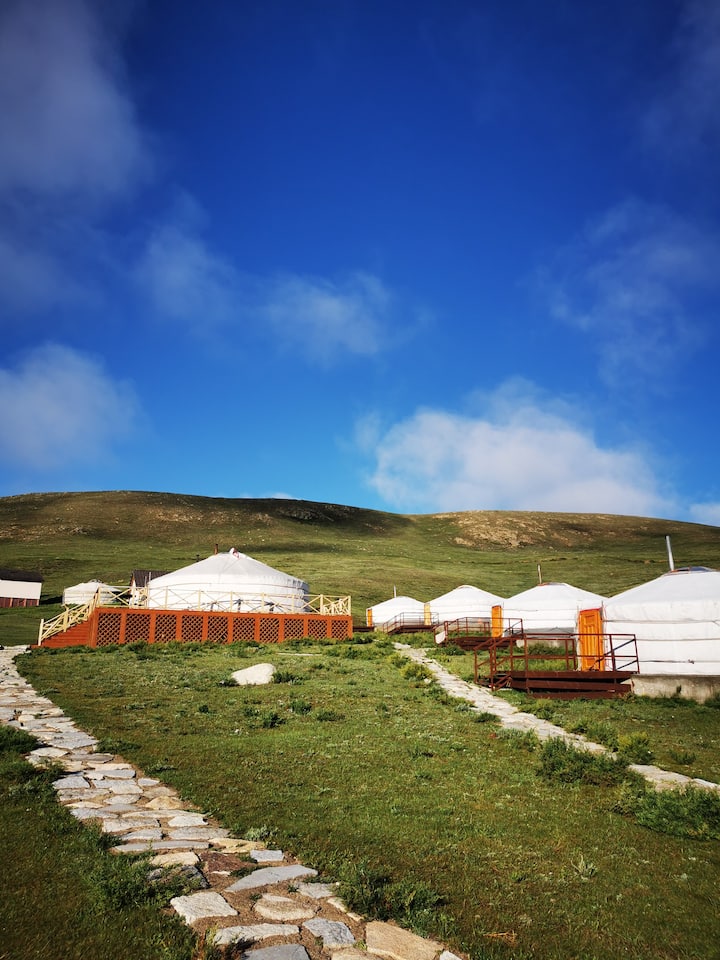The photograph showcases a picturesque grassy hillside under a vast, bright blue sky dotted with white, puffy clouds. Dominating the scene are several distinctive white domed buildings, each with orange doorways, reminiscent of drum-shaped tents or triangular forms that taper inward. The buildings are adorned with white antennas sticking out from the top. Intersecting the green field are stone cobblestone paths that wind up the hill. On the right, one path leads to a series of white domed structures, each with brown stairs and bright orange doors, recurring deeper into the scene. On the left, a larger set of burnt orange stairs, bordered by an off-white railing, ascends to another similar domed building. The paths and buildings rest on wooden bases, enhancing the quaint yet modern charm of the image.